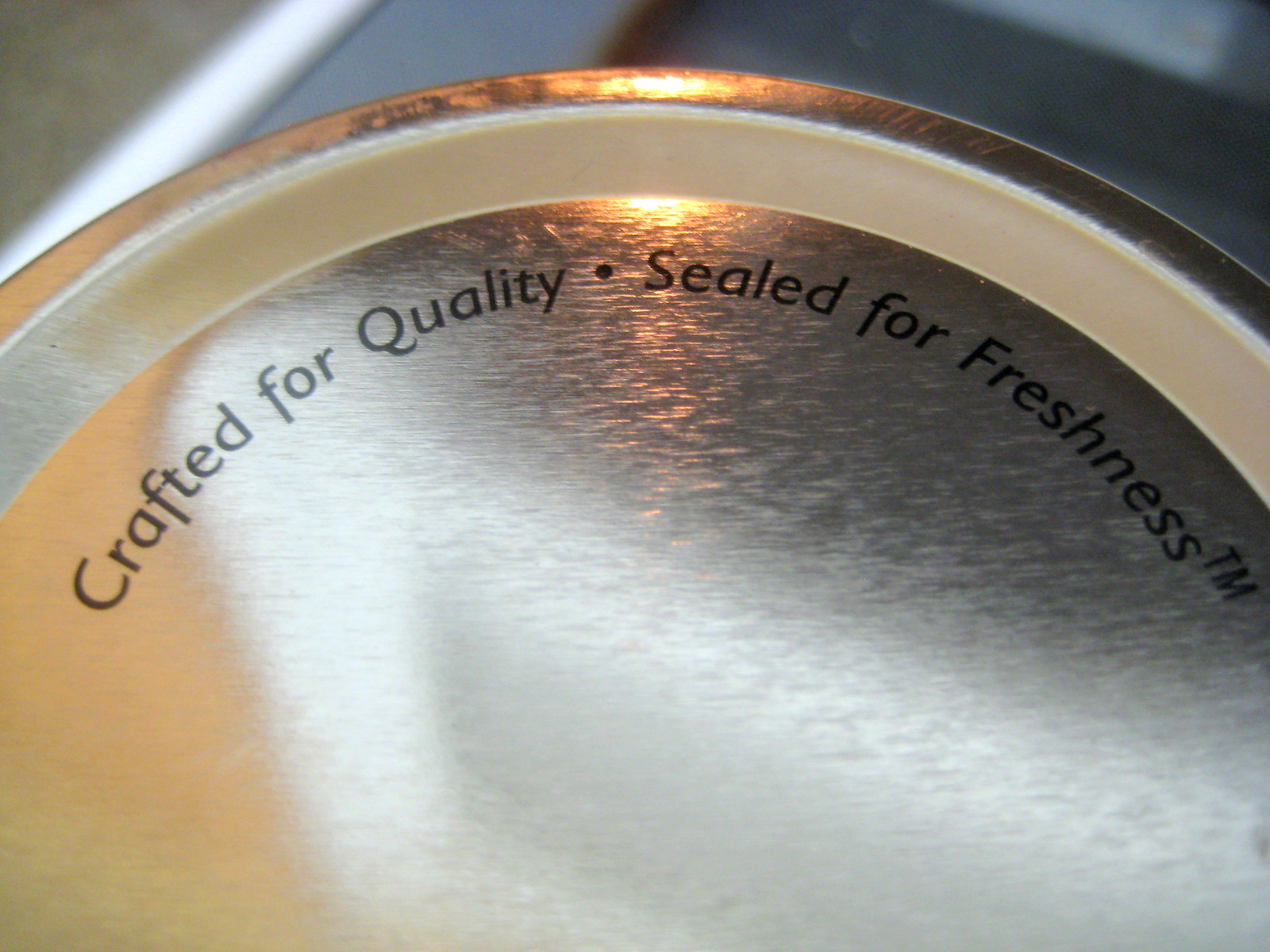The image showcases a close-up of a silver, shiny lid or seal typically used for a food container, with reflective properties capturing light from above. The metallic surface of the lid, which could be aluminium foil, is adorned with easy-to-read, solid black text that says, "Crafted for Quality, Sealed for Freshness TM." The wording suggests that this cover is designed to maintain the freshness of its contents, implying the item is likely related to food or a perishable product. The background is blurred, showing indistinct elements that might be a gray table and a tan floor or wall, making it difficult to discern specific surroundings. The object is partially cut off in the photo, but the visible portion indicates a rounded, container-like structure.